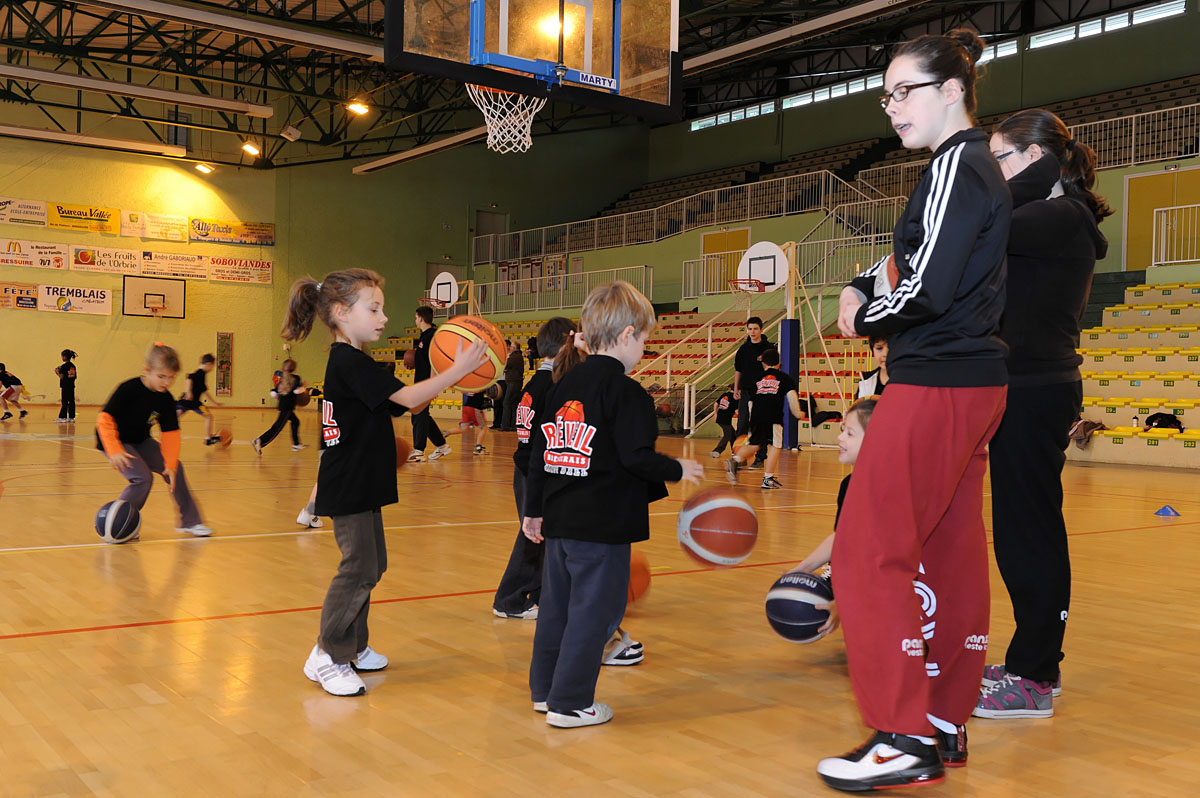In this landscape-oriented color photograph of an interior gymnasium, a bustling scene unfolds as many young children engage in a lively and somewhat disorganized basketball activity. Most of the children, who appear to be around six or seven years old, are dressed in matching black t-shirts that feature a graphic design on the back, possibly containing French text bordered in white with a basketball graphic above it. They are paired with long gray pants and sneakers. Boys and girls alike are scattered across the gym floor, each interacting with multiple basketballs, practicing dribbling techniques. The gym is equipped with several smaller basketball goals along the side near the empty bleachers, adding to the lively atmosphere.

At the right side of the image, two adult women are actively involved in directing the children. The woman in the foreground, with her hair up, is dressed in a long-sleeve black jacket, red athletic pants, and white sneakers. Another woman, also with her hair up, stands behind her in a black sweatshirt and long pants. Their attentive engagement suggests they might be coaching or supervising the kids. Additional adults can be seen in the background, further reinforcing the structured yet chaotic nature of the learning environment. The detailed photograph captures the essence of a busy, instructional setting within a gymnasium, providing a vivid snapshot of youth in action and the guiding hands nurturing their efforts.